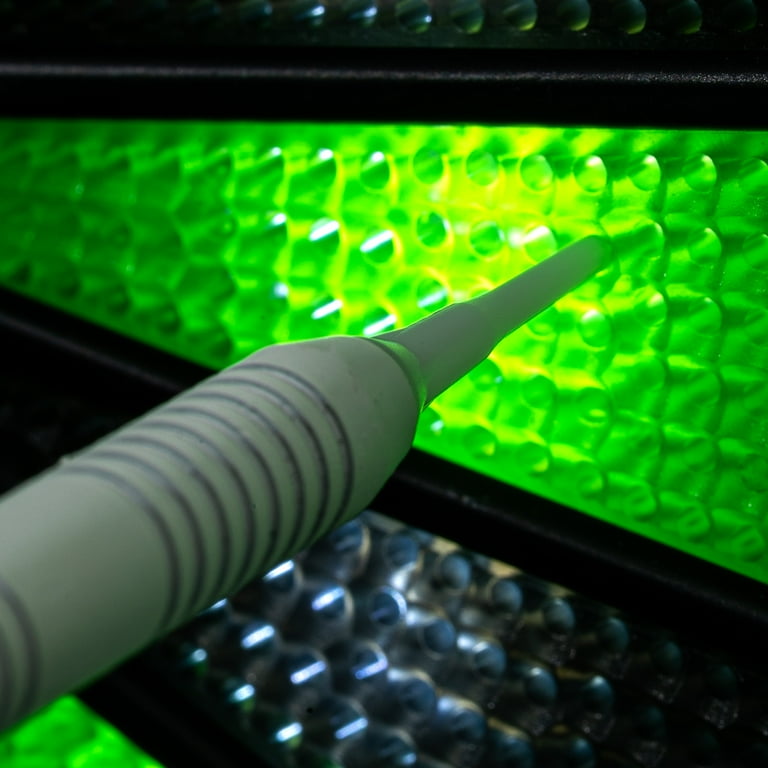This close-up photograph features a pointed gray stylus tool, possibly made or coated in plastic, with silvery gray ridges that are slightly dirty with dark spots. The tool protrudes diagonally from the left side of the image, with its tip inserted into a fluorescent green, gel-like surface marked by organized holes. This green surface features a bright mottled pattern of light extending from the right to the upper left of the frame, creating a visually striking backdrop against the tool. Surrounding this lit area, there are black rectangles at the top and bottom of the frame. Below the green surface, there's a dark gray unilluminated layer with a similar texture, and faintly visible in the bottom corner, an additional layer is lit green again. The leftmost side and the top and bottom of the image are slightly blurred, emphasizing the central focus on the stylus and the vibrant green, hole-pocked gel.